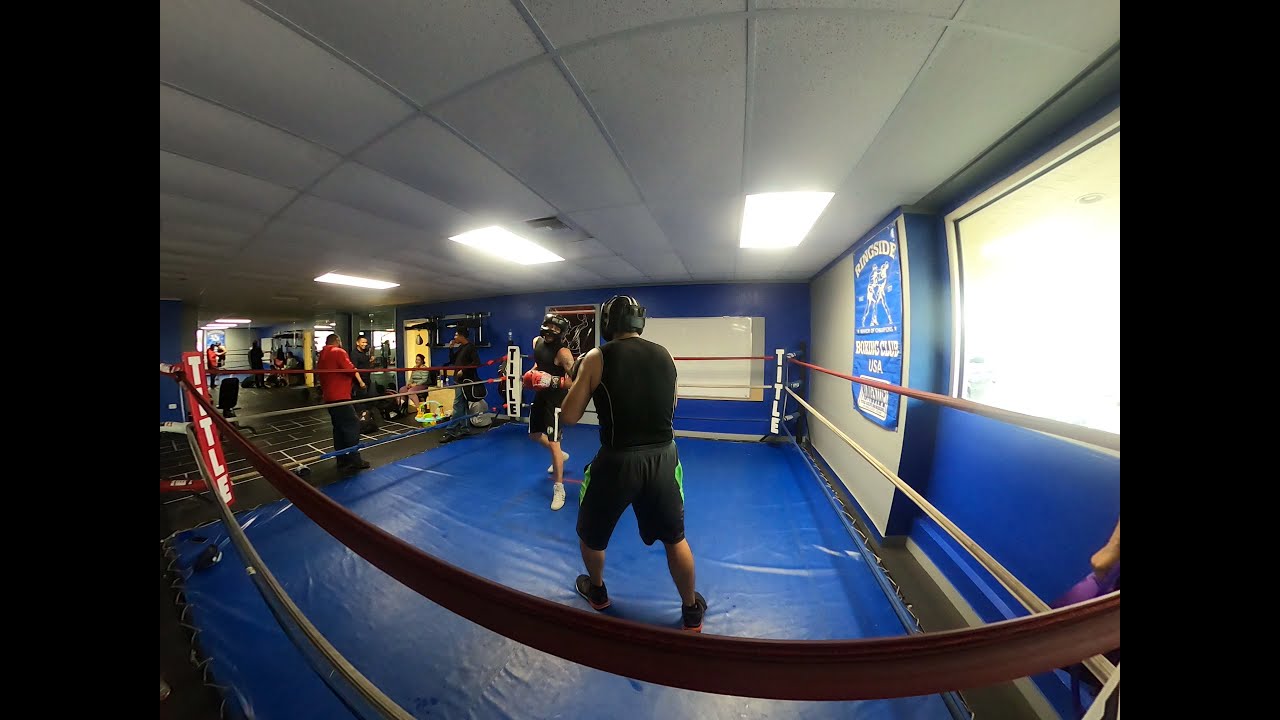In this photograph of an indoor boxing gym, the main focus is a boxing ring with a blue mat and boundary ropes that alternate between red and white colors. Inside the ring, two boxers are actively engaged in a match. Both athletes are dressed in sleeveless black shirts and black shorts; one pair of shorts features green stripes while the other has white stripes. They are also wearing dark-colored helmets for protection. One boxer is equipped with red boxing gloves, and their sneakers differ in color—one boxer has dark sneakers while the other sports white ones. Surrounding the ring, several people can be seen conversing, adding to the lively atmosphere. The gym features a white ceiling with bright rectangular fluorescent lights. The walls are blue and white and adorned with posters, including a prominent blue and white sign and a banner with white font on a red background, possibly indicating a match or the gym's name. To the left and right sides of the image, two vertical black strips frame the scene. Additionally, there's a man in a red shirt and black pants outside the ring, along with a few more people scattered in the background.